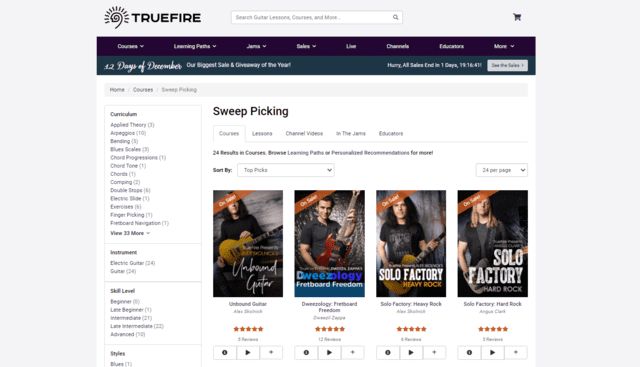This rectangular image, oriented horizontally, features a prominent gray border on the left and right side, with a thinner gray border at the top. At the very top center, the text "TrueFire" is displayed in dark blue or black lettering. The top right corner of the image includes a search box followed by a cart symbol.

Directly below this, a blue border spans the width of the image, displaying the labels “Courses,” “Learning,” and “Pass,” along with an additional, hard-to-read word in small print. Beneath the blue border, a turquoise border contains more features, including another search box located on the far right.

The main content area below these borders features the title "Sweet Picking" and displays several images of people playing the guitar, suggesting a focus on guitar instruction. On the left side, a vertical column lists various words, seemingly detailing a curriculum or menu that extends the full height of the image. Although the text is small and difficult to read, the top word appears to be "Curriculum,” indicating the content is likely educational material aimed at individuals learning to play the guitar.